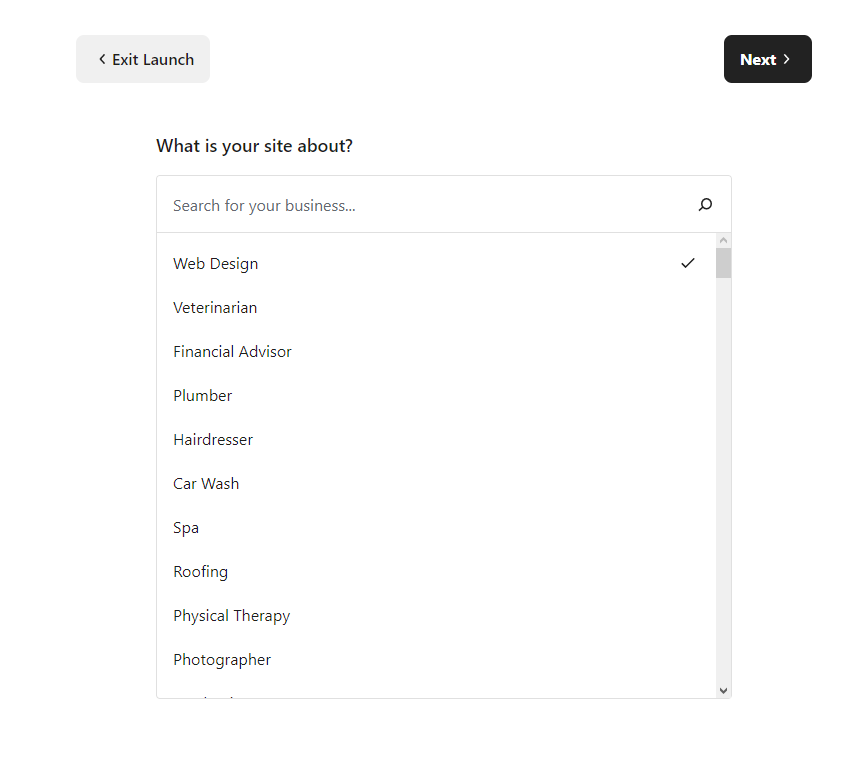The image features a user interface presented on a white background. At the top, there is a soft-edged, rounded rectangular button in gray that reads "Exit Launch" in black capital letters ("E" and "L" both capitalized), with a left-pointing arrow adjacent to it. Toward the right, another rounded rectangular button appears, this time in black, containing the word "NEXT" in white capital letters, with a right-pointing arrow.

Beneath these buttons, the text "What is your site about?" is displayed in bold black print, followed by a search bar below it. Inside the search bar, the placeholder text reads "Search for your business..." accompanied by a magnifying glass icon on the right end.

Below the search bar, a list of categorized options is neatly arranged in a column. The categories are as follows:
1. Web Design (with a check mark on the right side)
2. Veterinarian
3. Financial Advisor
4. Plumber
5. Hairdresser
6. Car Wash
7. Spa
8. Roofing
9. Physical Therapy
10. Photographer

On the right side of the list, there is a thin gray scrollbar, enabling users to scroll through the list. The design elements and interactive components suggest a clean, user-friendly interface for selecting business types during a site setup process.